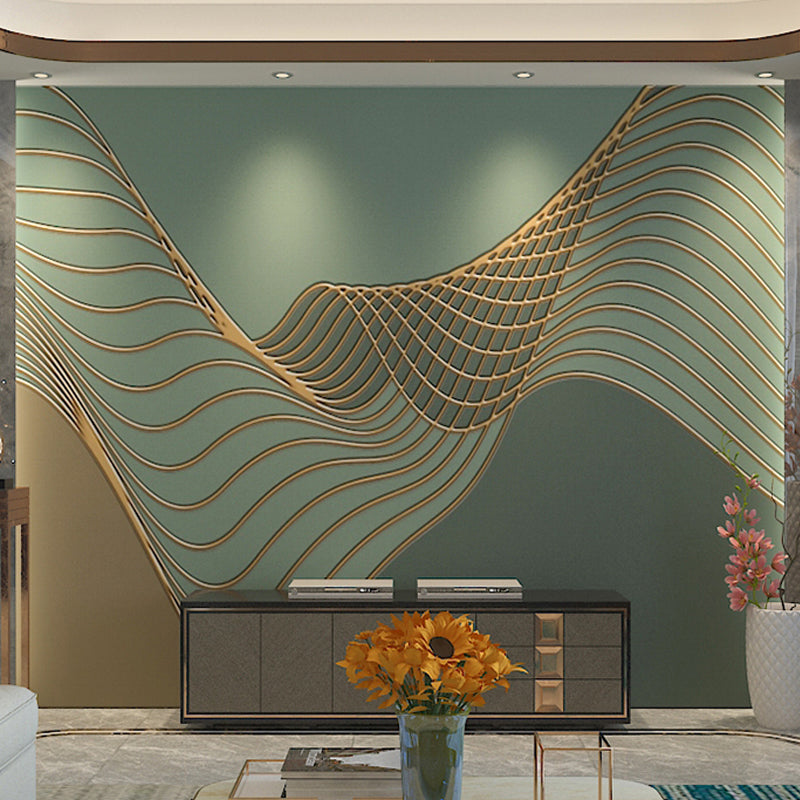This photograph captures a modern, sophisticated reception area in what appears to be a hotel lobby or a high-end business office. The focal point is a stylish brown dresser cabinet with four drawers, positioned against a dual-toned wall—half green and half brown/mauve—adorned with an intricate gold pattern. The cabinet hosts two thin electronic devices, possibly music amplifiers. Four ceiling-mounted spotlights highlight the gold pattern, adding to the room's elegant ambiance. Adjacent to this setup are two tan-colored couches placed on a tan and white marble floor, creating a comfortable waiting space. A glass coffee table between the couches holds a striking blue metal vase filled with artificial gold sunflowers, alongside a stack of thick magazines, contributing further to the refined yet welcoming atmosphere.